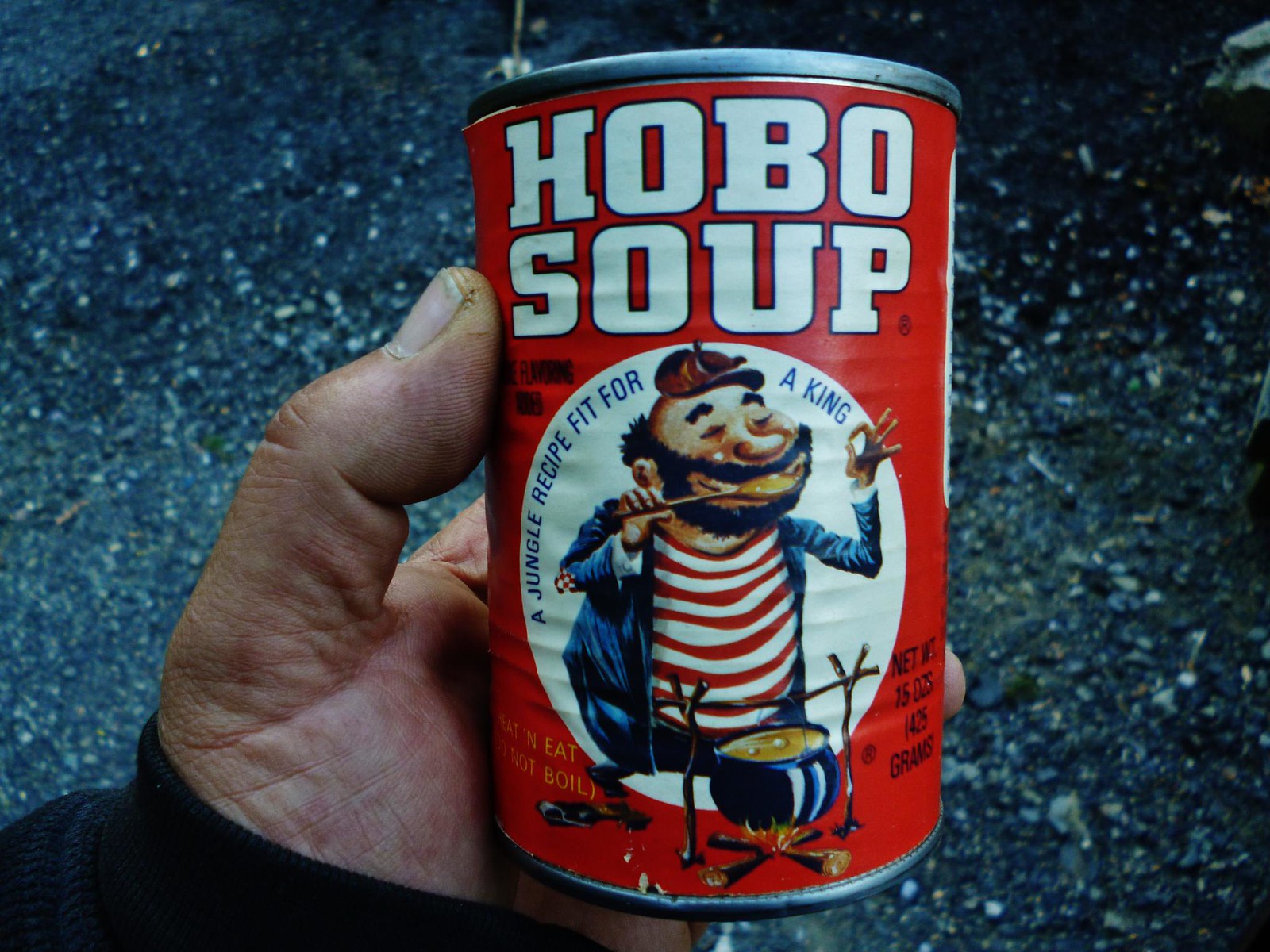In this close-up photograph, a weathered and partially dirt-stained hand, clad in a blue sleeve, firmly grasps a vibrant red can of soup labeled "Hobo Soup." The sleeve covers a portion of the hand, which is the sole focus along with the can. The rugged backdrop consists entirely of small, thin rocks and gravel in a mix of gray, blue, and white tones, laid over what appears to be concrete. The can itself features whimsical and nostalgic artwork: a man in a white and red striped shirt, complete with a hat, is depicted licking a spoon as he tends to a cauldron suspended over a fire by two sticks. The label reads, "Hobo Soup - A Jungle Recipe Fit for a King," adding an adventurous and hearty touch to the scene.